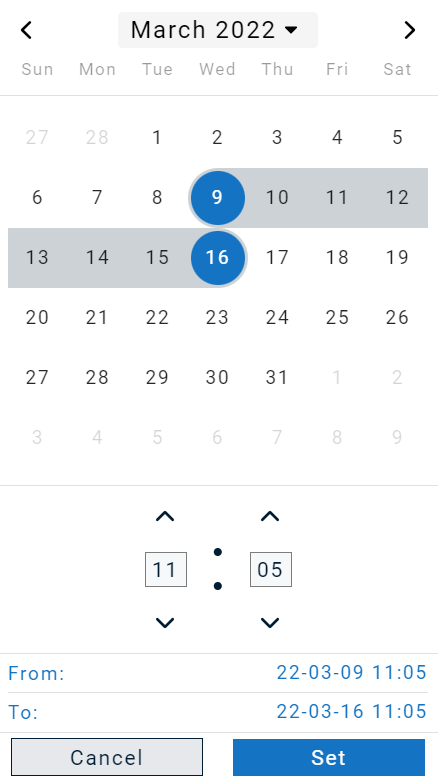The image showcases a cell phone screen displaying a calendar application set to March 2022. At the top of the screen, navigation arrows are visible, allowing the user to move back to February or forward to April. The days of the week are listed in abbreviated form: Sun, Mon, Tue, Wed, Thu, Fri, Sat.

In the calendar grid, dates from the previous month, February 27 and 28, appear in a lighter shade. The current month's dates are fully visible, ranging from 1 to 31. Additionally, the first few days of April (1 and 2) are included, continuing into the following week up to April 9.

A specific range of dates, from March 9 to March 16, is highlighted in gray, with the numbers 9 and 16 encircled in blue. Towards the bottom, there are control options featuring up and down arrows next to the numbers '11' and '05'. There are also "Cancel" and "Set" buttons available for user interaction.